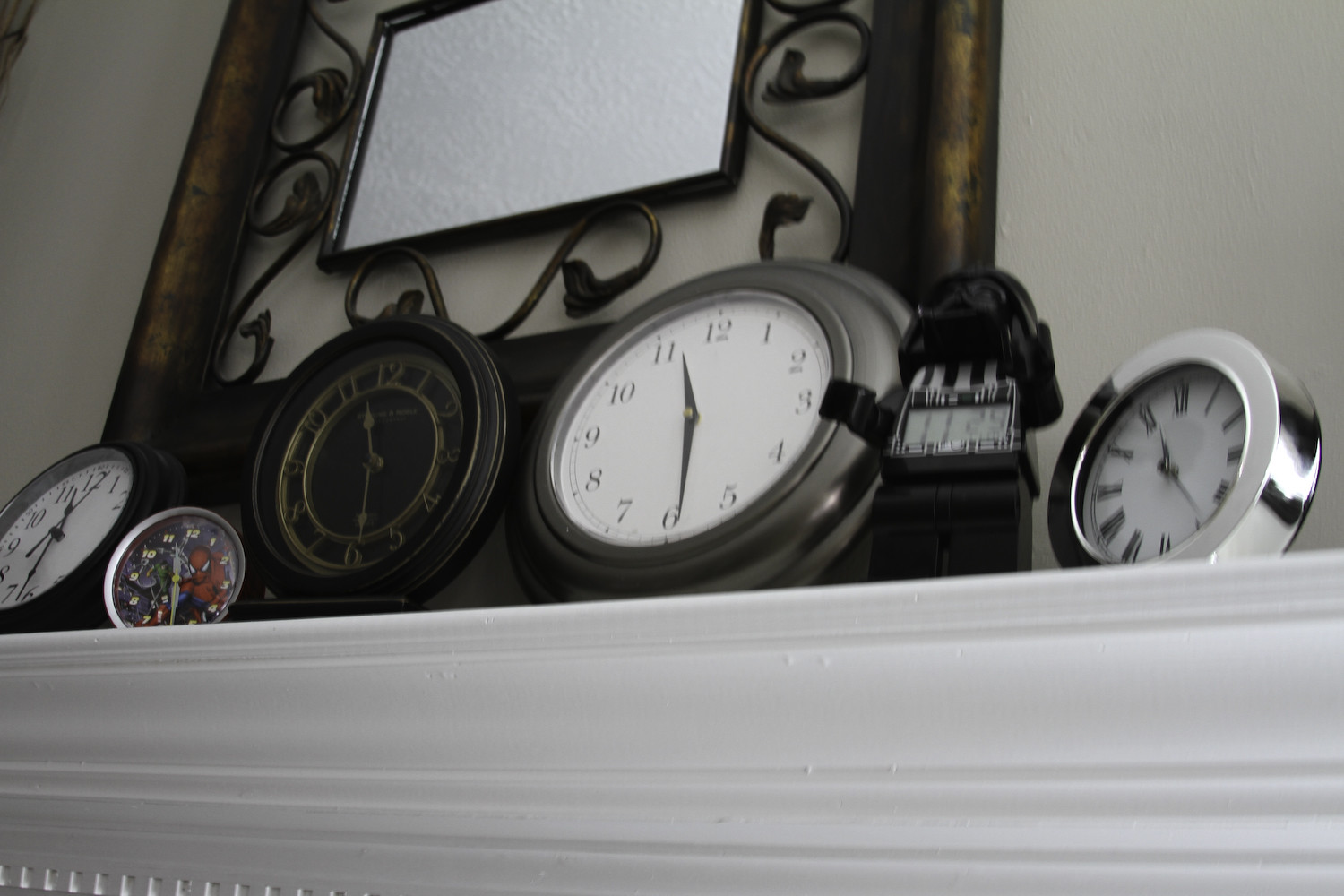The image captures a detailed snapshot of a white mantle above a fireplace, reminiscent of crown molding with a glossy finish. Resting on the mantle are six distinct clocks, all set around 11:30, with one slightly off at 11:25. From left to right, the first clock is round with a brown rim and a white face, featuring long black hands. Next, there's a smaller Spider-Man-themed clock, silver-rimmed with a black face and gold numbers. The third clock, larger and wood-rimmed, sports goldish numbers and hands. Following this is a slightly bigger clock with a silver frame, white face, and black hands. To its right stands a black Darth Vader figurine resembling a Lego character, featuring a digital clock display. The last clock on the far right has a silver frame, a white face with black Roman numerals, and is slightly turned. Above the mantle hangs a central mirror with brown squiggly designs extending outward, framed by a brown border that continues off the top edges of the image.